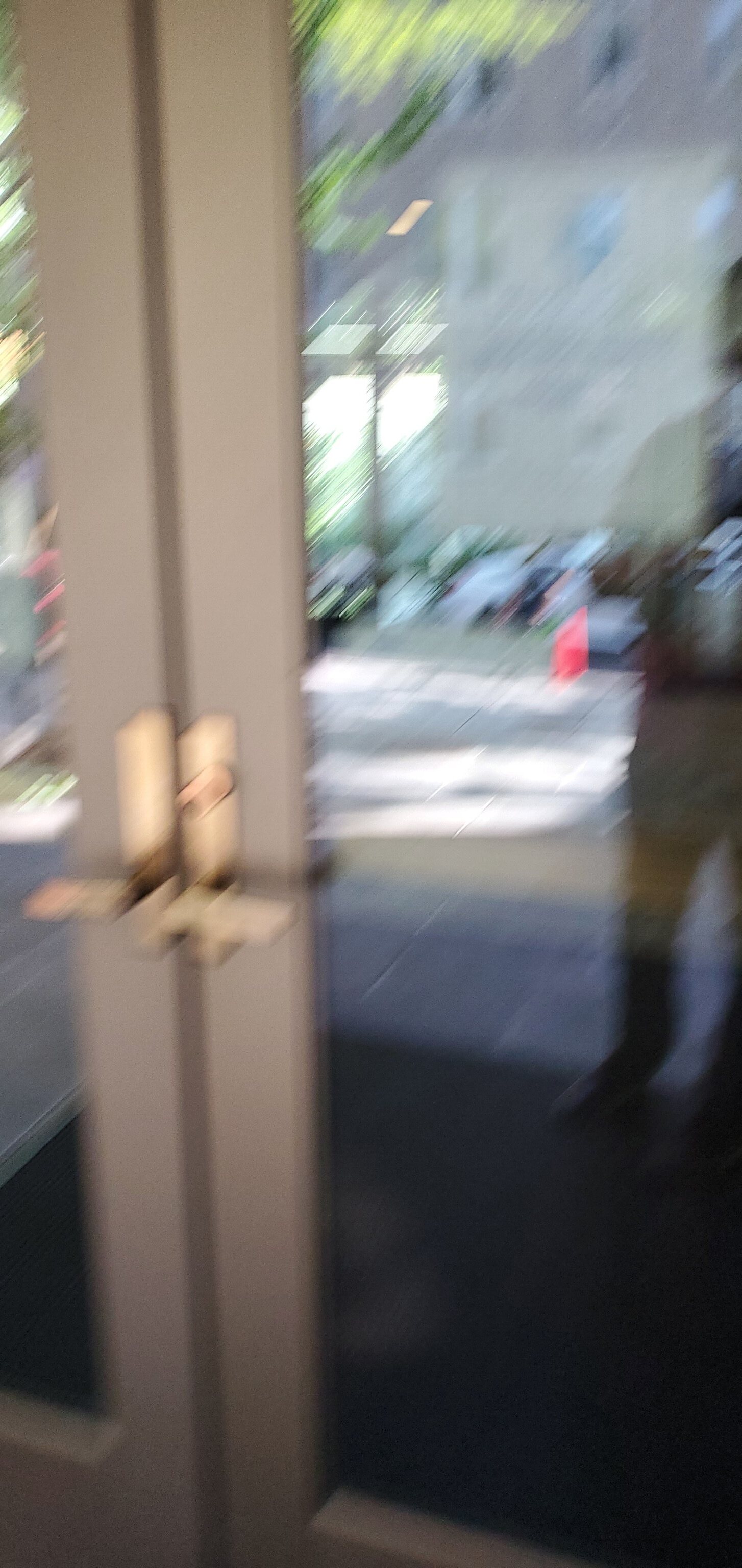The image showcases a pair of French doors with a brown wooden frame and gold handles, slightly off-center to the left of the photo. Although the picture is quite blurry, the glass doors reflect sunlight and hint at an outdoor scene with a roadway and possibly a fence in the background. There’s a faint, barely discernible figure standing in front of the doors, their image mirrored in the glass.